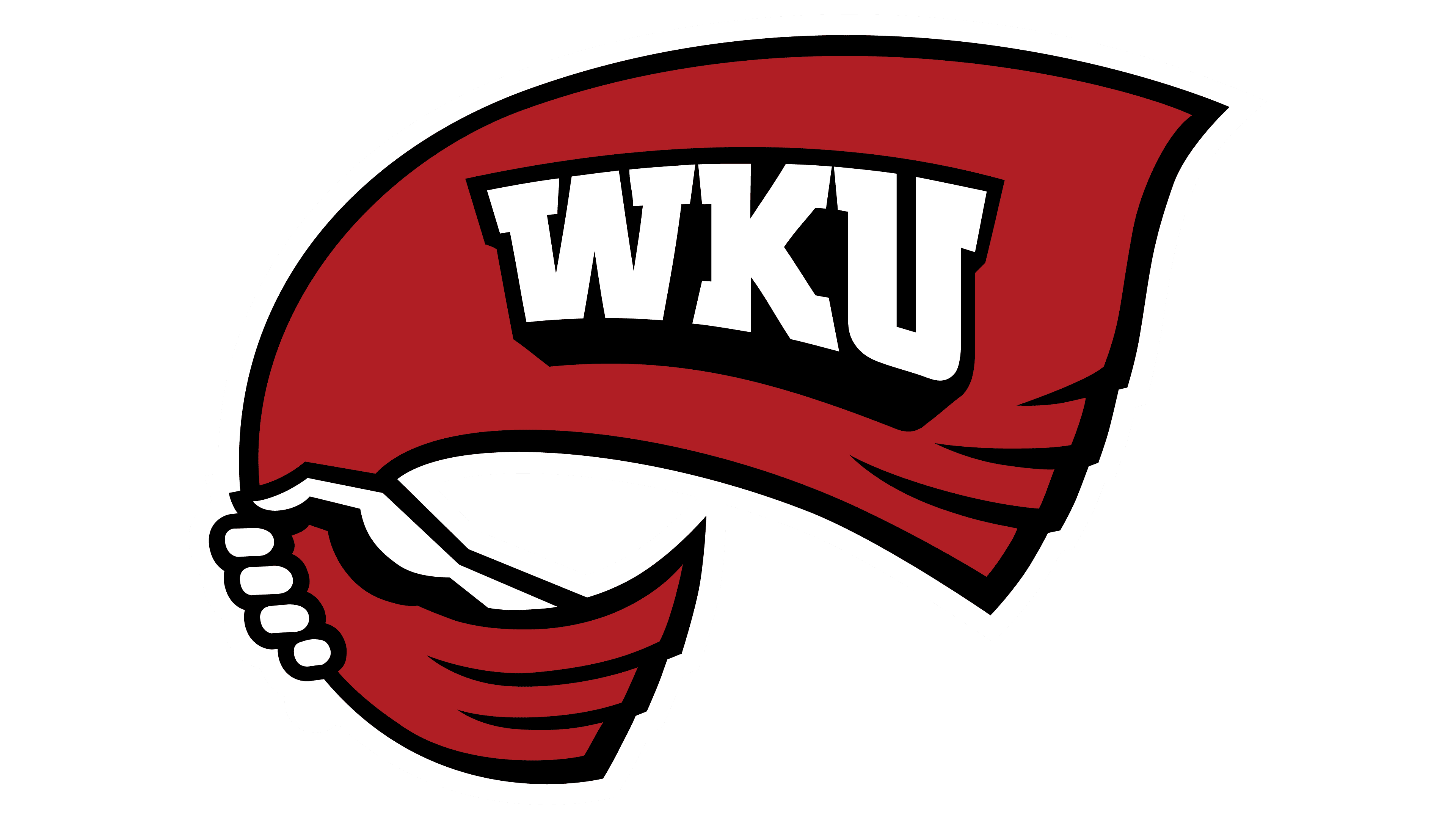The image is a striking cartoonish logo for Western Kentucky University, characterized by bold use of red, white, and black. On a white background, a thick black border outlines the entire design, which features a red fabric—resembling a scarf or banner—gripped firmly by a right hand. The hand, detailed with a black outline, shows the thumb and palm clasping the top of the fabric, while the four fingers curl around the back, making a fist. The fabric appears to be trailing through the fist and folding at the bottom right, suggesting movement. Prominently displayed in the center of the red fabric are the initials "WKU" in bold, white uppercase letters, set against a black rectangular backdrop. This dynamic and impactful logo encapsulates the spirit of Western Kentucky University, located in Bowling Green, Kentucky.